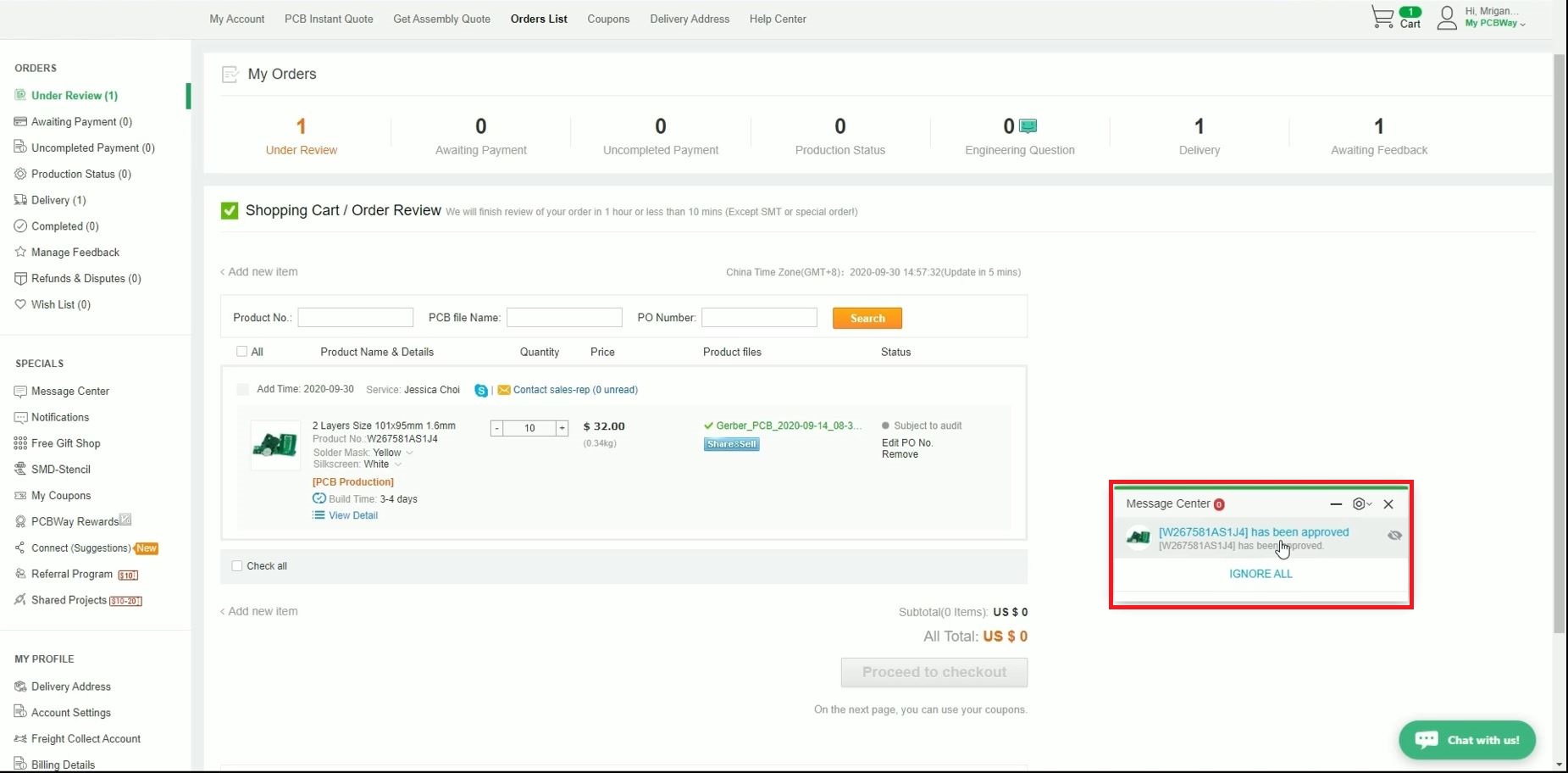The screenshot captures the interface of an account management page. At the top-left corner, 'My Account' is prominently displayed. Below it, there are multiple tabs labeled with three-word phrases, which are difficult to read due to their small size. The legible tabs include 'Orders List,' which is highlighted in bold, black text, while the other tabs, such as 'Compare,' 'Coupons,' 'Dietary Actions,' and 'Help Center,' appear in a lighter, gray text.

On the top-right side, there's an icon of a shopping cart with a green circular badge displaying a white number, either '5' or '1,' which is hard to distinguish. Next to it, a greeting message reads, "Hi, Megan," followed by various order statuses:

- My Orders: 1
- Under Review: 0
- Awaiting Payment: 0
- Unaccepted Payment: 0
- Pending Status or Production Status: 0
- Expecting (unspecified status): 1
- Delivery Awaiting Feedback: 1

At the bottom of the page, there is a green rectangle button with the white text, "Chat with Us," indicating an option for customer support.